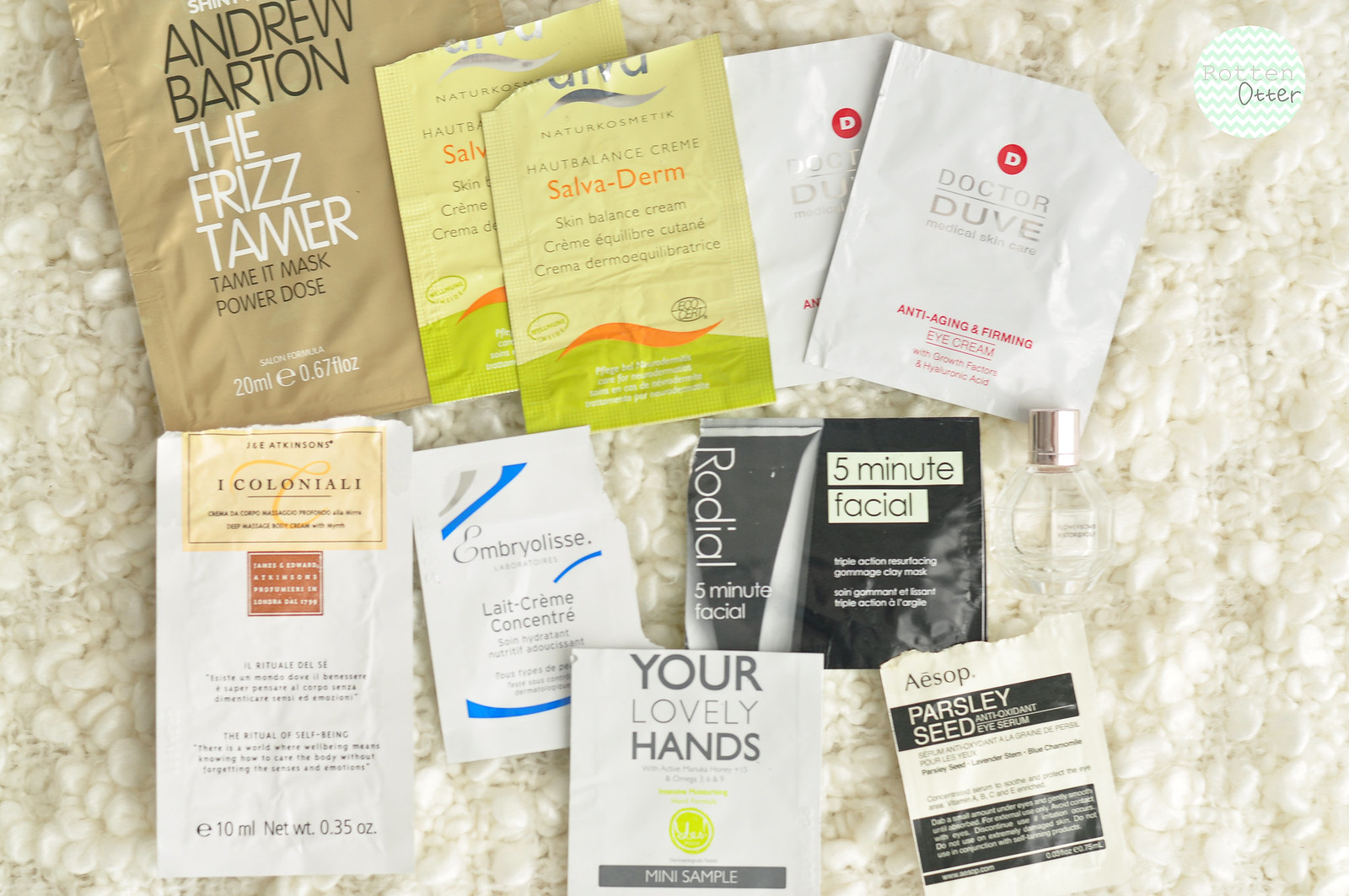The image showcases an array of sampled product packets meticulously collected and arranged, presumably by an avid skincare enthusiast or a conscientious reviewer. These samples, spanning a variety of creams and masks, lie flattened on a knitted, textured bedspread of off-white wool, adorned with loops or knots for added visual interest. 

In the top left, we observe a beige packet from Andrew Barton labeled "Tame It Mask Powder Dose," a frizz-taming hair treatment. Adjacent to it are two packets from Nature Remedic, featuring a skin balancing cream with light green and beige coloring. Below these, two white packets with silver and red text from Dr. Duva promise anti-aging and firming benefits. 

Further down lies a sample from E.Coloniali, a brand associated with Atkinson's, likely offering a facial cream. Nearby, a small white packet with gray and blue prints bears the name Embryolisse and identifies itself as "Le Creme Concentré," a nourishing milk cream for the face. Next in line, a five-minute facial from Rodial, presented in both black and white packets, promises quick skincare efficacy. 

At the bottom, a sample labeled "Your Lovely Hands Mini Sample" features gray writing and a distinctive yellow logo. The collection concludes with a packet of Aesop's antioxidant eye cream, formulated with parsley seeds.

In the top right corner of the image, a watermark featuring a circle with squiggly lines and the text "Rotten Otter" suggests the identity of the collector, potentially hinting at an impending review or comprehensive analysis of these products.